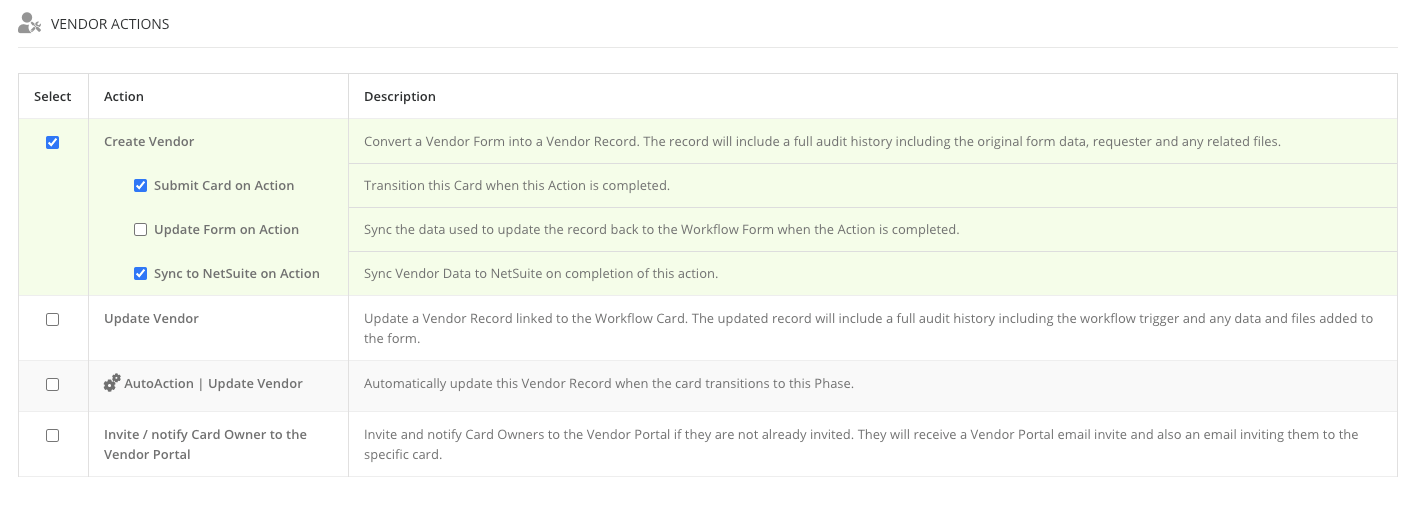The image appears to be a screenshot from a software interface related to vendor actions. In the upper left corner, there is a gray user icon. To its right, slightly blurred, is the text "Vendor Actions" in black. Below this header, there is a light gray outlined box sectioned into columns labeled "Select," "Action," and "Description."

Within the box, the first four entries are highlighted in green, indicating selection. The specific actions shown include "Create Vendor," "Submit Card," and "Sync to [something]," each paired with their corresponding actions. Beneath these, three entries are not highlighted, which are "Update Vendor," "Auto Action Update Vendor," and "Notify Card Owner to the Vendor Portal," indicating they are not selected.